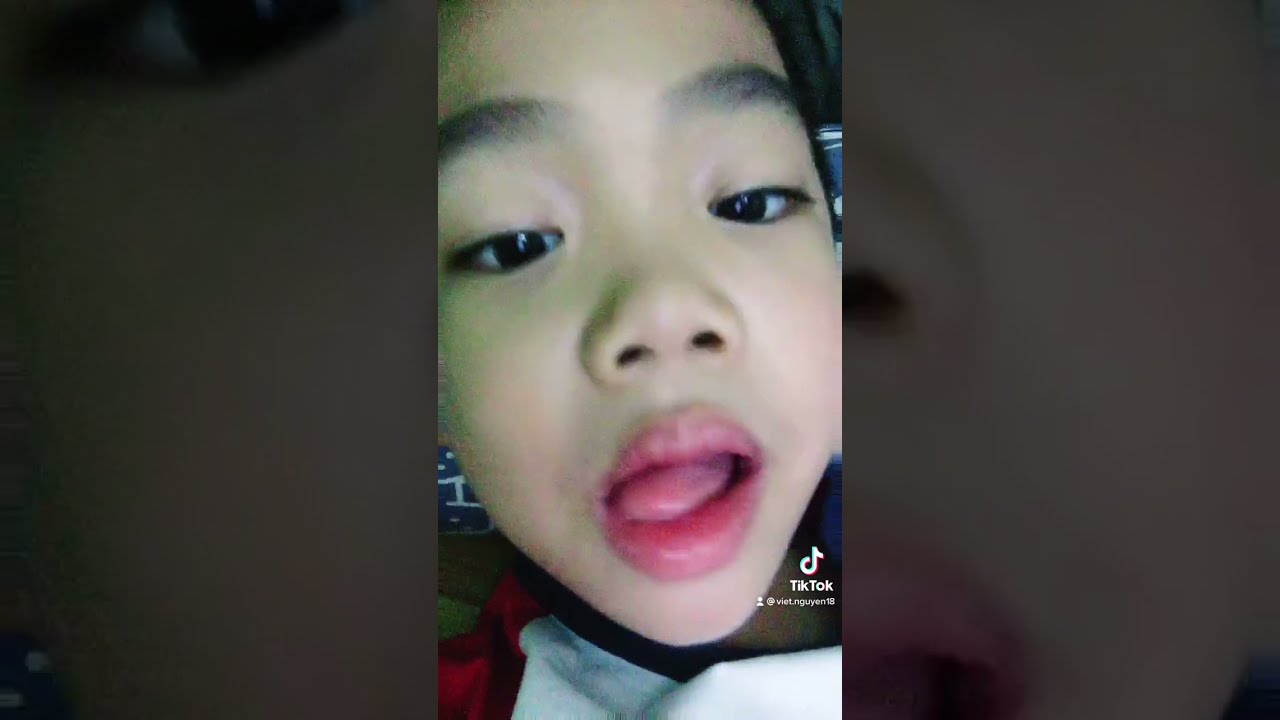The image is a close-up selfie taken from a TikTok video, identified by the TikTok logo and text at the bottom right corner that reads '@Viet.Nguyen'. The slightly blurry and low-light shot focuses on the face of a young girl, who appears to be of Asian descent, with dark eyes, black eyebrows, and pink lips. She has her mouth open with her tongue pushed toward the left side, partially sticking out. Her skin has a dark tan complexion. The girl is wearing a shirt that has both blue and red colors, although it's not very visible as her face dominates the image. The background shows indistinct objects in various colors. The overall atmosphere feels a bit hazy around the edges, adding to the impression of a casual and spontaneous selfie moment.